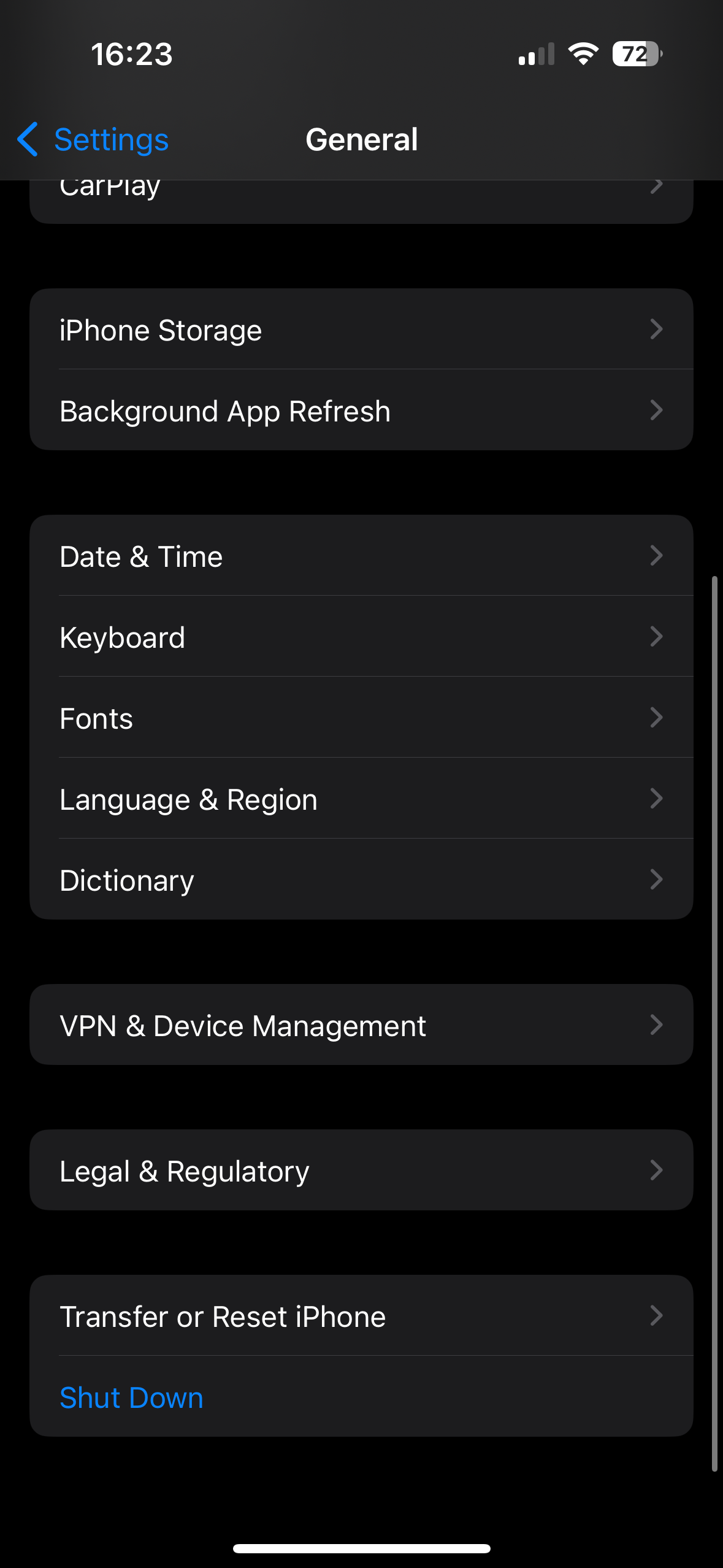This image is a screenshot from a smartphone displaying a section of the device's Settings menu. The time at the top reads 16:23, and the top-right corner shows various icons including signal coverage, Wi-Fi connectivity, and a battery indicator at 72%. The image features a black background with the header "Settings" in blue text at the top, accompanied by a left-pointing blue arrow.

Below this header, the menu title "General" is displayed in white text. The screenshot captures a list of options available under this menu: "CarPlay," "iPhone Storage," "Background App Refresh," "Date and Time," "Keyboard," "Fonts," "Language and Region," "Dictionary," "VPN and Device Management," "Legal and Regulatory," and "Transfer or Reset Phone." The final option, "Shutdown," is uniquely highlighted in blue text.

The image is portrait-oriented, meaning it is taller than it is wide. A white horizontal line appears at the very bottom center of the image, presumably indicating an area to swipe up to return to the home screen. The screenshot is void of any photographic or illustrative elements, strictly featuring textual content. There are no living beings or natural elements depicted in the screenshot.